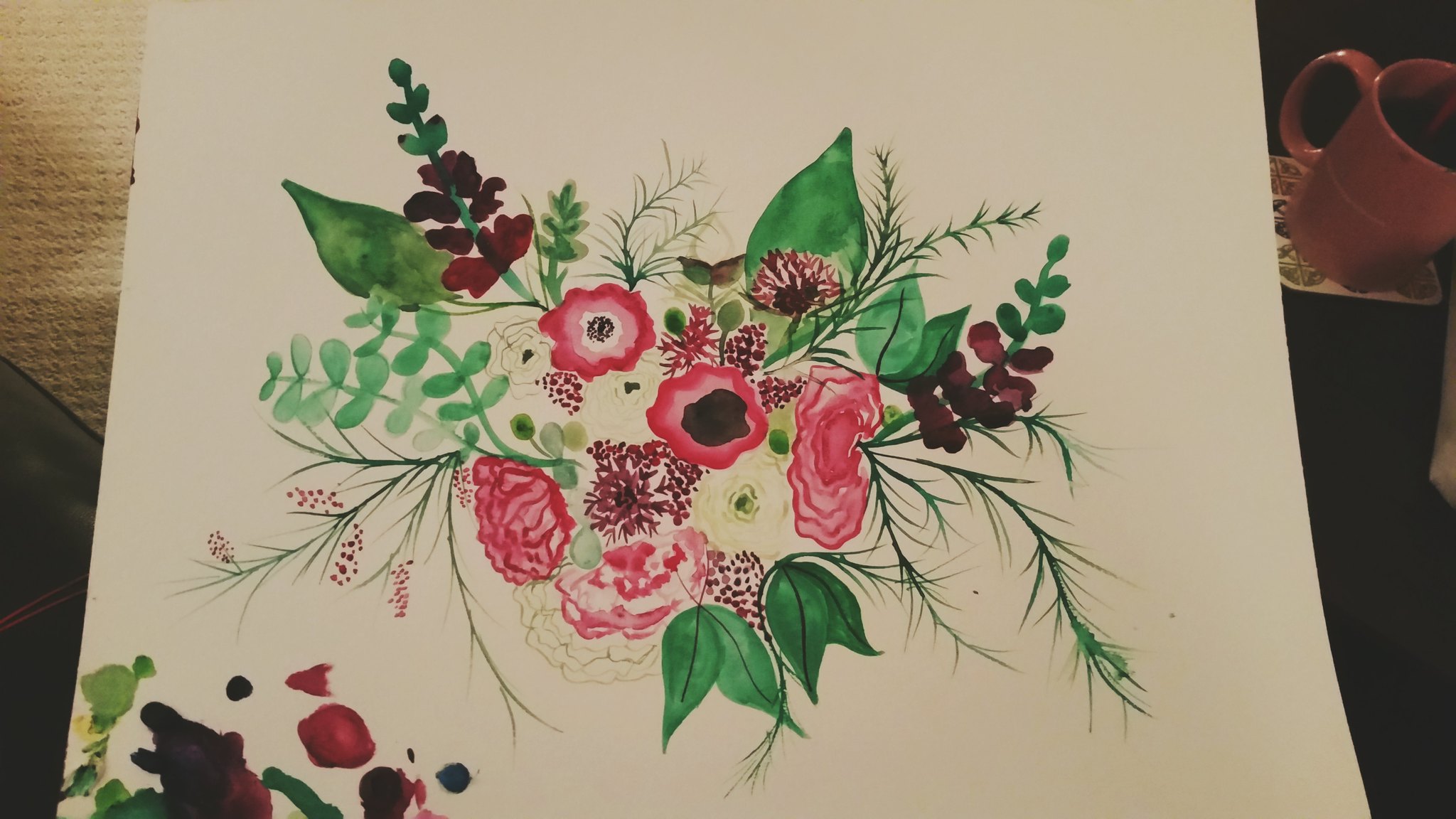The image showcases a detailed watercolor painting on white paper, placed on a table. On the right side of the table, there's a clay-colored coffee cup resting on a mat. The left side of the image reveals the brown edge of the table, and above it, a light tan cloth.

The watercolor painting itself is a floral design, featuring vibrant pink and white flowers at its center. One of the flowers boasts a large brown center, while another has a white and brown center. Surrounding the flowers are various green leaves, including both large and small types, as well as thin greenery and foliage adorned with berries. In the bottom left-hand corner of the painting, there are intricate ink marks in shades of red, light green, and dark green, adding a unique touch to the artwork.